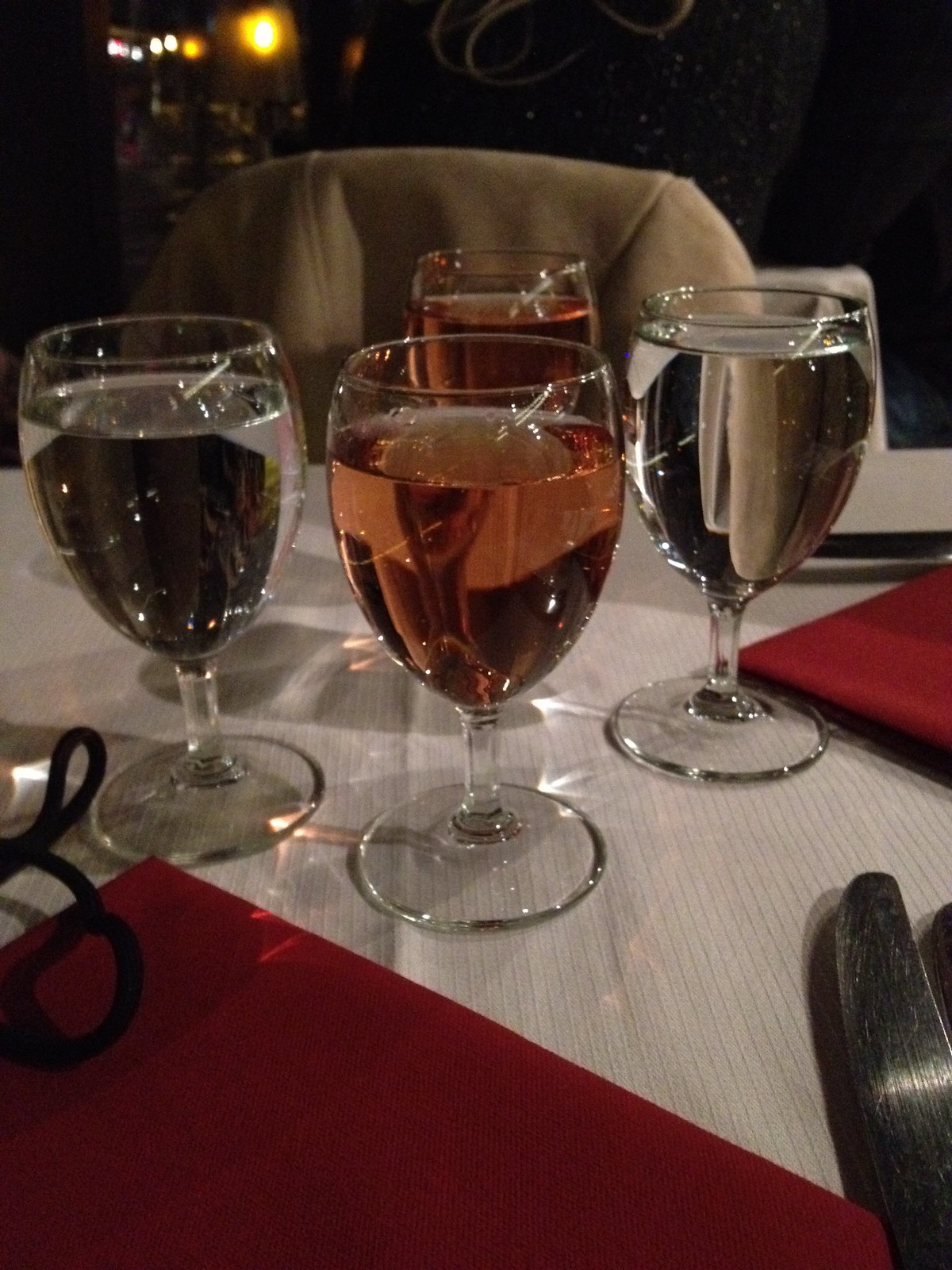In this dimly lit restaurant, the photo captures a cozy and atmospheric dining table adorned with a white tablecloth. There are four identical wine glasses arranged in a neat fashion. Two of these glasses, positioned front and back center, contain a light rosé-colored wine, while the other two, placed on the left and right, hold clear water. The table is set with red linen napkins and a silver butter knife is visible towards the bottom right of the image. A red menu lies on the table, along with a black cord looping nearby. In the background, a gray or tan jacket is draped over the back of a chair, adding to the casual elegance of the setting. The room is dark with only a few distant lights visible in the upper left corner, casting gentle sparkles on the glassware. This intimate scene speaks to a moment of quiet dining, rich with ambiance.